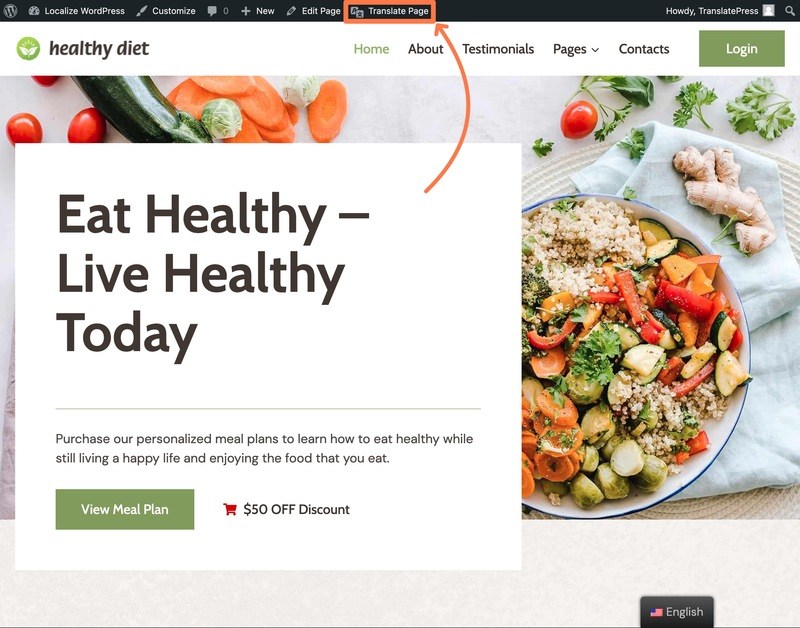This screenshot captures the homepage of a website called "Healthy Diet." At the top of the page, there is a black text header that reads "Healthy Diet," flanked on the right by a navigation menu that includes categories such as Home, About, Testimonials, Pages, and Contacts. Adjacent to this menu is a green rectangular box with white text that says "Login."

Below the header is a partial image of a vibrant, healthful bowl of food. The bowl includes an assortment of grains, zucchini, red peppers, Brussels sprouts, carrots, and some type of greens, all presented on a white napkin. Unpeeled pieces of ginger are strategically placed around the bowl. The background of the image features an array of miscellaneous vegetables like carrots, tomatoes, zucchini, Brussels sprouts, and parsley, adding to the visual appeal.

To the left of this centerpiece, a white box with black text boldly declares, "Eat Healthy, Live Healthy Today." An eye-catching orange arrow extends from this box to the top of the page, pointing to an option labeled "Translate Page."

Below this box, an encouraging message reads, "Purchase our personalized meal plans to learn how to eat healthy while still living a happy life and enjoying the food you eat." Just beneath this text is another green rectangular box with white text, inviting viewers to "View Meal Plan." To the right of this invitation, a special offer states "$50 off discount," accompanied by a small red shopping cart icon. This well-structured layout appeals to visitors by combining visual elements with essential information, promoting a holistic approach to healthy living.